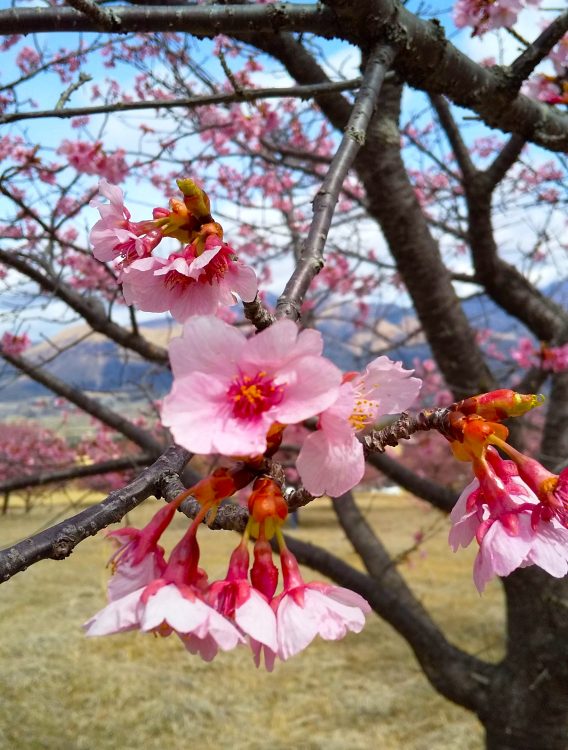This stunning photograph captures a close-up of vibrant cherry blossom flowers in full bloom on a branch of a dark-barked tree. The exquisite pink blossoms, each with a dark red center and visible pollen, are prominently displayed against a backdrop of a pale blue sky. The scene also includes rolling hills with patches of brown and green, suggesting a mixture of meadows and scattered trees. The grass beneath the tree and in the surrounding meadow is a hay-like tan color, indicating early spring before the full greening. Off in the distance, similar blossoming trees can be seen, adding depth to this serene orchard landscape. Wispy white clouds float in the sky, completing this picturesque and tranquil outdoor scene.